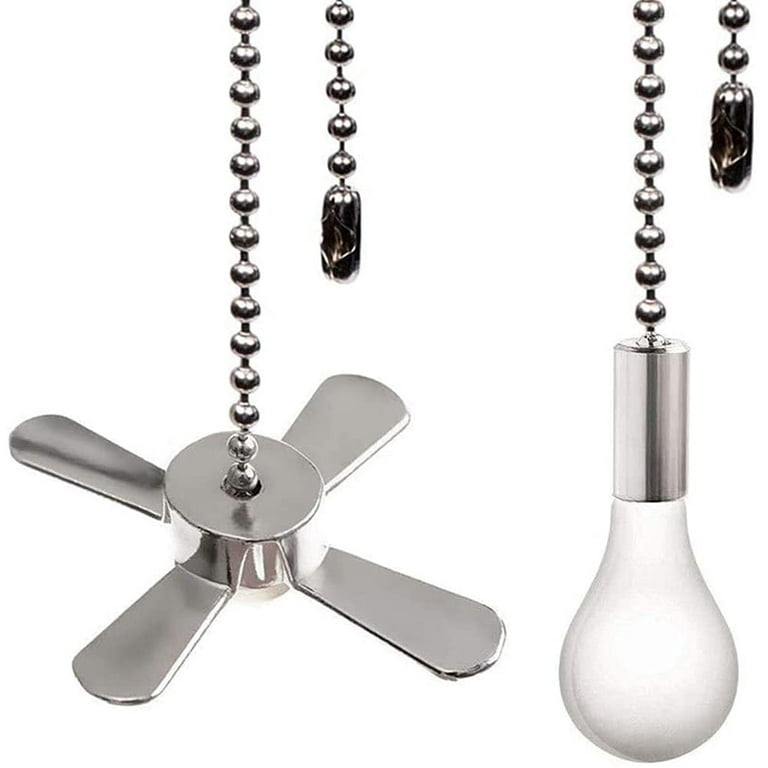The image showcases a scene featuring a light bulb and a mini fan. On the right side of the image, a white light bulb is hanging from a metal chain composed of small metallic balls. This chain connects to a metal base, which supports the light bulb. Adjacent to the chain, towards the top right corner, there is a small metal tassel, which functions as a pull chain to turn the light on or off.

On the left side of the image, another metal chain identical in style to the one on the right extends further downward and connects to a small silver metal fan with four blades. Above this fan, slightly to the top right, there is another pull chain with a metal tassel, which is noticeably longer than the tassel connected to the light bulb. This second tassel likely serves to control the fan's operation. The overall scene captures the intricate details of these connected fixtures, highlighting their metallic textures and functional design elements.